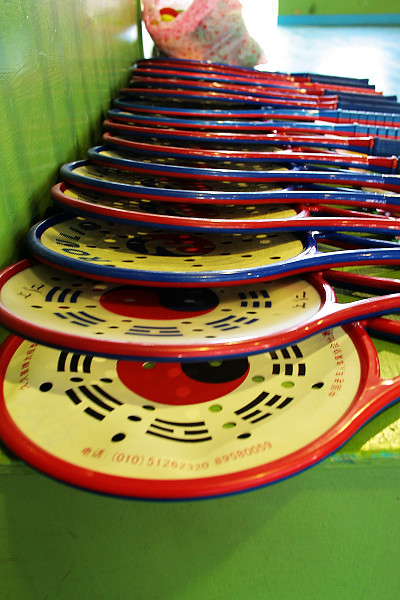The image depicts a stack of colorful sports rackets with red and blue metal edges and a prominent yellow circular center. Each racket features a flexible, solid surface adorned with perforations in various circular and rectangular shapes, forming a design that includes a distinctive red and black yin-yang symbol. The rackets bear writing in an Asian language and have blurred numbers around the edges. They are neatly arranged in a row on a green wooden shelf, leaning against a green backdrop. In the background, a floral-patterned bag filled with an assortment of multicolored items, including red, yellow, green, and blue balls, is visible. The floor transitions from a bright green in the foreground to a vibrant teal in the background.